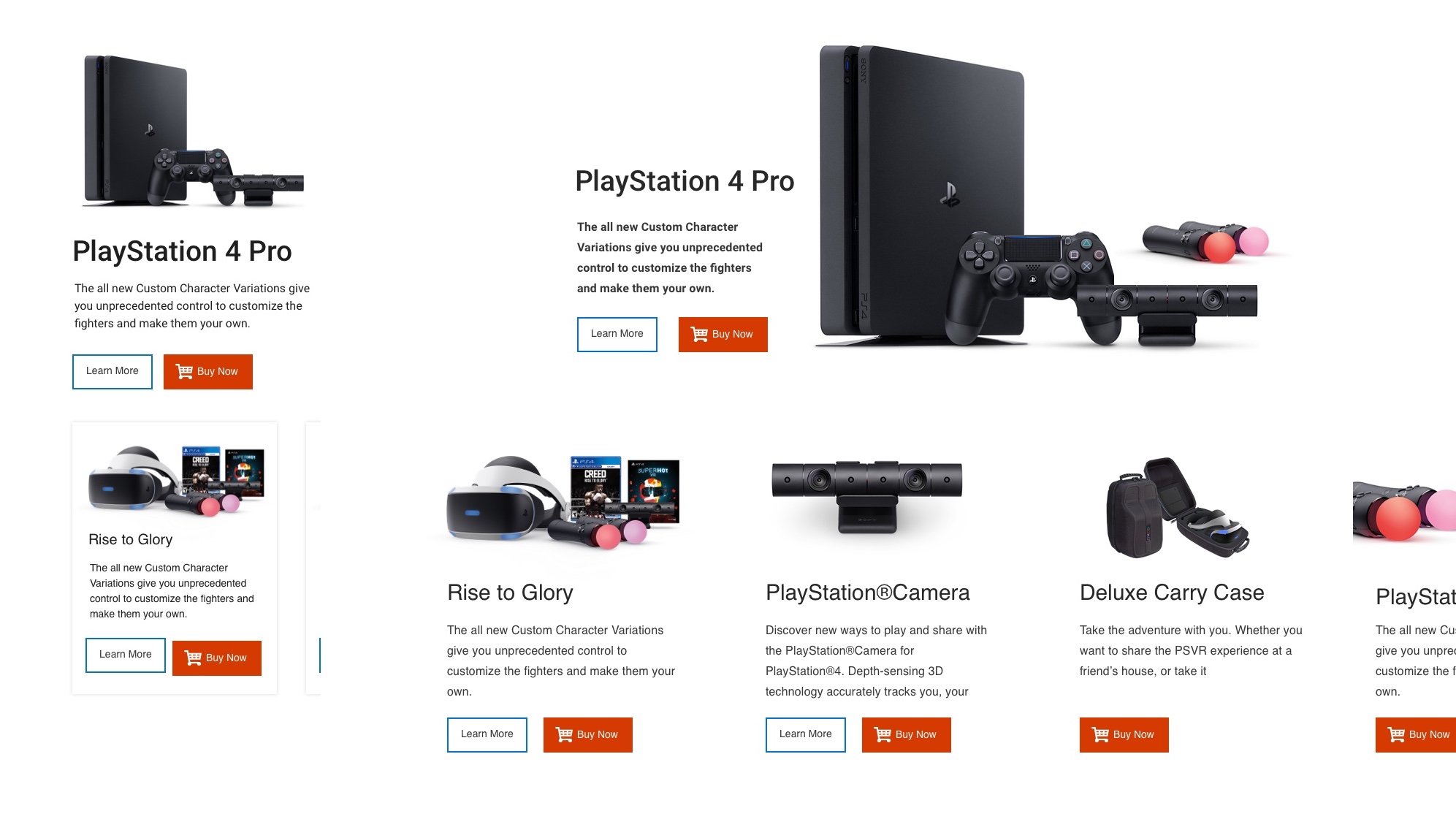The image is a promotional screenshot divided into two columns, depicting a comparison between a compact and a detailed version of a PlayStation 4 Pro advertisement. 

The left column, resembling the potential size of a cell phone portrait, displays the PlayStation 4 Pro console. Below it, there is a brief descriptive text followed by two buttons: a clear green button labeled "Learn More" and a red button with a shopping cart icon labeled "Buy Now." Additionally, above the description, there is a monitor and a PlayStation holder. The tagline "Rise to Glory with the all-new custom character" is prominently displayed above the buttons.

The right column features a more expansive landscape version of the same advertisement. Here, the description of the PlayStation 4 Pro is larger and situated on the right side of the console image. The buttons "Learn More" and "Buy Now" are identical to their counterparts on the left. This detailed version also includes additional elements not seen on the left: a PlayStation camera, a deluxe carry case, and a partially visible section cut off at the edge, potentially showing more accessories. A striking red and pink handle-like object is also present next to the description in this column.

In summary, this image juxtaposes a concise mobile-friendly design with a comprehensive landscape layout, both promoting the PlayStation 4 Pro with consistent call-to-action buttons and enriched with extra details in the larger version.